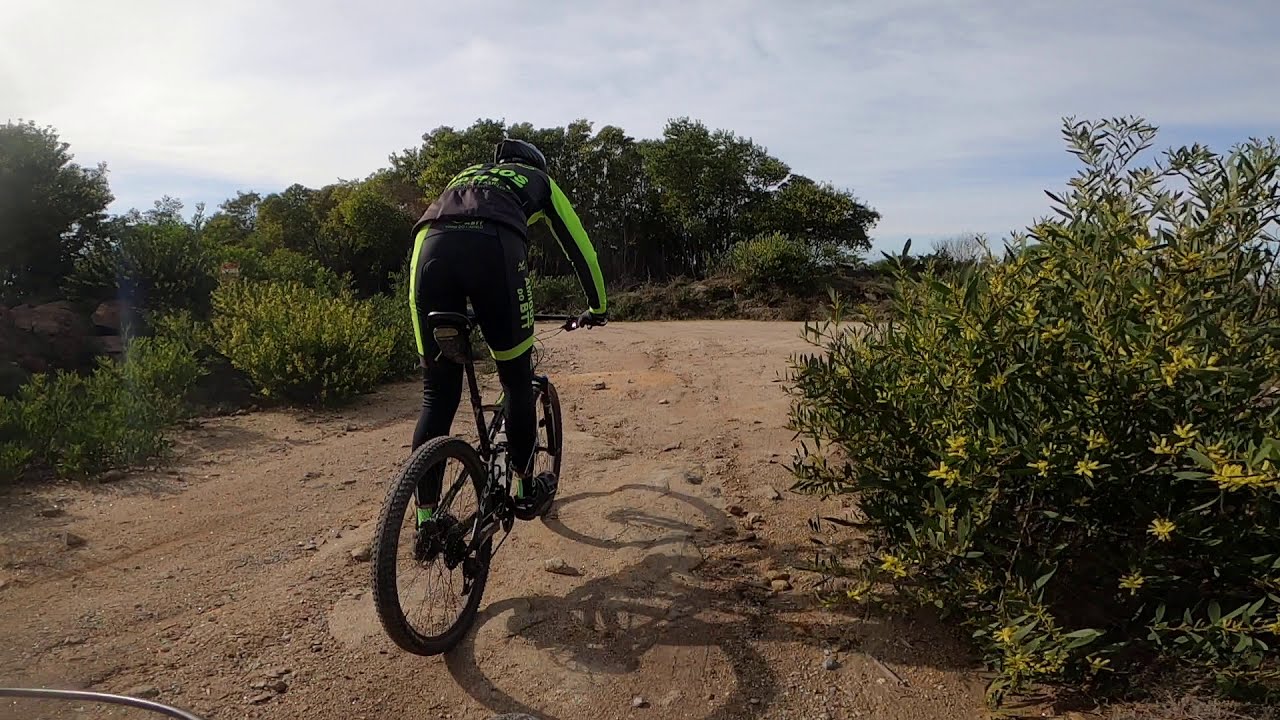In this photograph, we see a cyclist, predominantly positioned to the left, navigating up a small, brown dirt hill covered in pebbles and rocks. The cyclist is on a mountain bike equipped with off-road tires and is fully dressed in a green and black long-sleeve uniform, complemented by a helmet and hiking shoes. The path the cyclist is on is flanked by green shrubs, with some yellow flowers on the right side of the image, and a scattering of trees farther in the distance. The sky above is mostly cloudy, allowing some patches of blue to peek through, while the sunlight casts the shadow of the rider and bike to the right. This dynamic outdoor scene conveys the thrill and adventure of mountain biking.